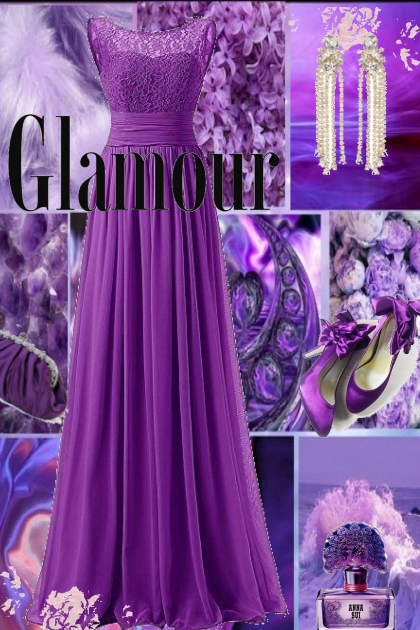The image is a vertical, rectangular collage predominantly shaded in various hues of purple, conveying a luxurious and high-end aesthetic. Central to the image is an elegant, sleeveless purple gown with a long skirt and lacy detailing at the top, draped across the upper portion, leaning to the left. Behind this gown, the background features an artistic blend of purples, resembling clouds interspersed with faint floral elements. The word "Glamour" is prominently displayed in black letters in front of the dress. Surrounding the gown are smaller squares and rectangles of different shades of purple, showcasing high-end fashion items such as bottles of expensive perfume, intricate jewelry pieces like earrings and necklaces, and fashionable shoes. A particularly notable element to the right of the dress is a small rectangle featuring a golden arch against a purple backdrop, enhancing the opulent theme. The overall composition is a harmonious collage of fashionable and luxurious items, reflecting a sophisticated, glamorous vibe.